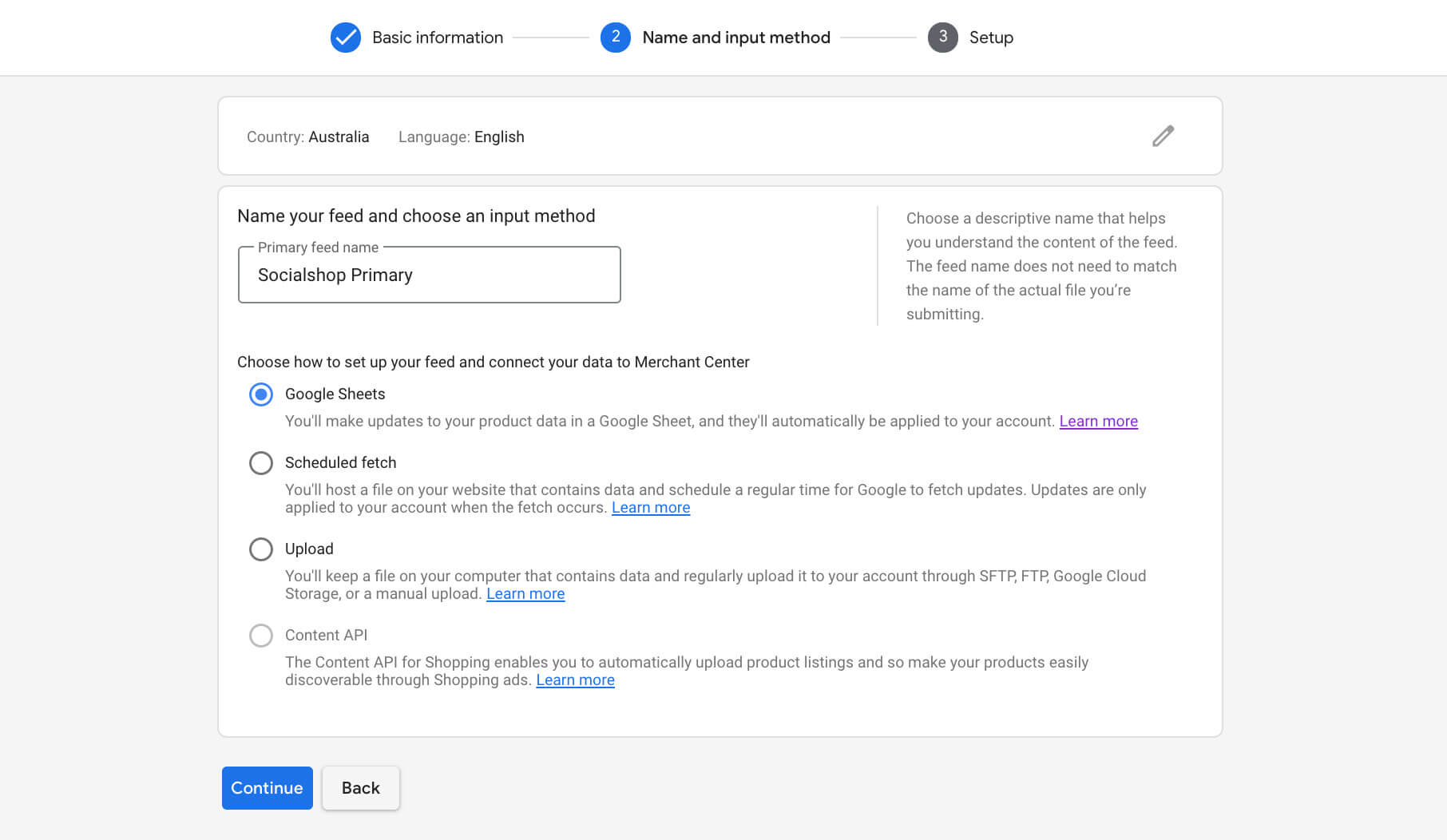The image is a screenshot featuring a user interface set against a white background. The header at the top of the screenshot reads "Basic Information," accompanied by a blue circle with a white checkmark inside it, situated to the left of the text.

Immediately below the header, the interface displays sections labeled "Name" and "Input Method," followed by another section titled "Setup." These are framed within the screenshot's design elements.

The next section has a light gray background and contains a white box. Inside this box, from left to right, the text denotes that the country is set to "Australia" and the language is set to "English."

Moving down, there is another white box with black text that instructs the user to "Name your feed and choose an input method." An open input field labeled "Social Shop Primary" is situated beneath these instructions. To the right of this input field, in smaller gray text, appears a note advising the user: "Choose a descriptive name that helps you understand the content of the feed. The feed name does not need to match the name of the actual file that you're submitting."

At the bottom left corner of this section, additional instructions prompt the user to "Choose how to set up your feed and connect your data to Merchant Center." Below these instructions, four options for data connection methods are listed: "Google Sheets," "Scheduled Fetch," "Upload," and "Content API."